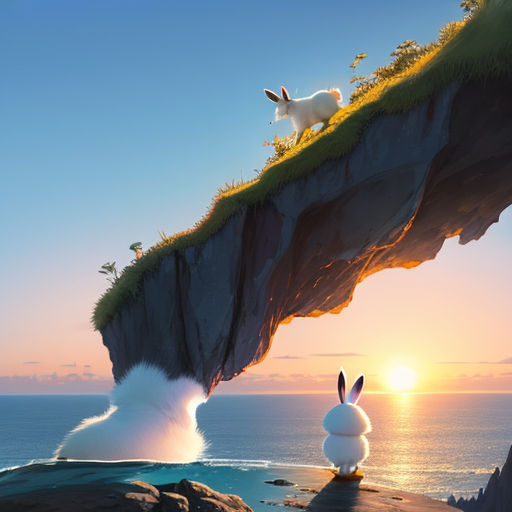The image is a square, computer-generated illustration of a fantasy scene featuring two white, rabbit-like creatures with pointy ears. The backdrop is a serene seascape with the sun, depicted as a light yellow circle, just above the water. The sky transitions from the yellow and pink hues around the sun to a clear blue as you move upward, with a horizontal layer of gray, feathery clouds midway.

In the foreground, rocky ground and brown rocks set the stage. A white bunny, standing upright and with its back to the viewer, gazes out at the sunset. Diagonally stretching from the upper right corner to the lower left, a piece of cliff covered in grass and possibly flowers or mushrooms juts out. Atop this cliff stands another bunny on all fours, angled downward as if it might fall. Between the cliff and the ocean, a white, ice-like object connects the cliff structure to the ground, enhancing the fantastical quality of the scene.